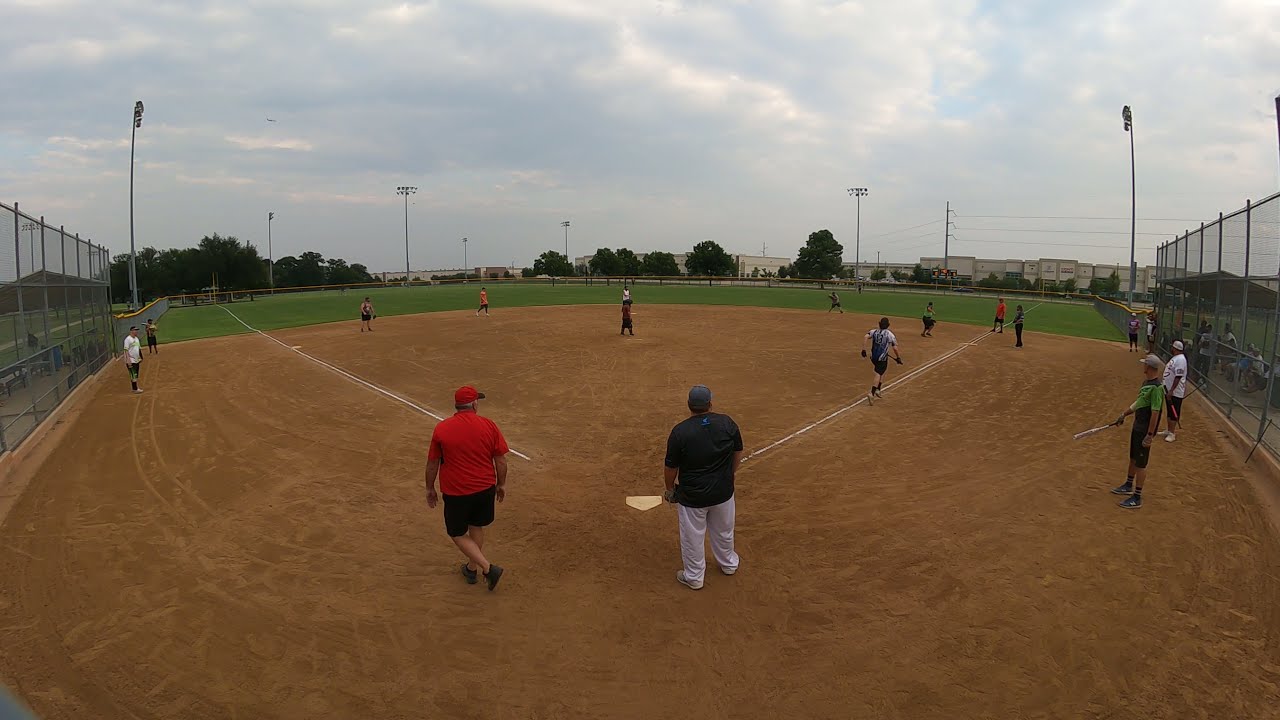The photograph captures an outdoor baseball game on an overcast day, taken from behind home plate. The sky is heavily clouded, and there are no signs of sunlight. Surrounding the field are six large banks of lights, currently turned off. The playing field itself is a typical baseball diamond, with dirt in the infield and lush grass in the outfield. A chain-link fence encircles the entire field, providing varying heights to protect spectators from stray balls.

In the foreground, the dirt infield features clearly visible white chalk lines, marking the first and third baselines and home plate. There is a player jogging toward first base, accompanied by a catcher in black gear and an umpire dressed in red standing nearby. Another player on deck can be seen swinging a bat. The outfield displays several tall green trees beyond the fence, adding a natural backdrop to the setting. 

Casually dressed players, identifiable neither by team colors nor specific uniforms, are sporadically positioned both in the infield and outfield. On either side of the diamond, nearer to home plate, there are higher chain-link fences likely intended to protect spectators, who can be seen gathered behind these barriers. The scene hints at a casual or older men's softball league, rather than a professional match.